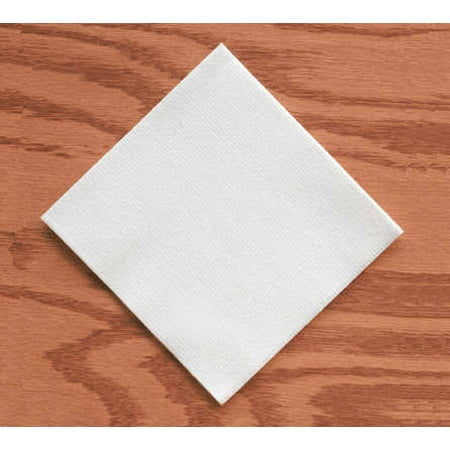The photograph features a simple yet striking composition of a single white square object, possibly a napkin, placed diagonally against a rich, horizontally grained wooden background. The wood, a seamless expanse of light to dark brown hues showcasing natural wavy patterns, contrasts vividly with the textured white cloth. The napkin is meticulously centered in the frame, arranged with its points perfectly aligned along the vertical and horizontal axes, creating a diamond shape. The lighting, subtly emanating from the top right, enhances the texture of both the wood and the napkin, adding depth to the stark, unadorned aesthetic of the scene.